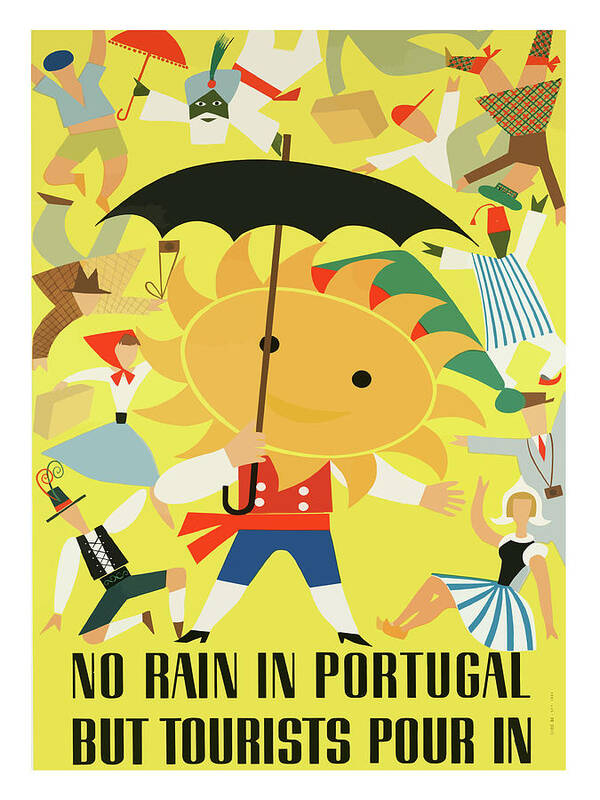The poster features a vibrant yellow background adorned with images of faceless figures dancing in traditional attire from various countries. The attire includes colorful dirndl-style dresses, peaked hats, clogs, vests, and short pants. At the center of the poster, a prominent figure with a sun-shaped face holds a black umbrella. Below this central figure, black text reads, "No rain in Portugal, but tourists pour in." The scene vividly depicts an array of national costumes, highlighting the diversity of cultural attire while emphasizing the allure of Portugal as a bustling tourist destination.